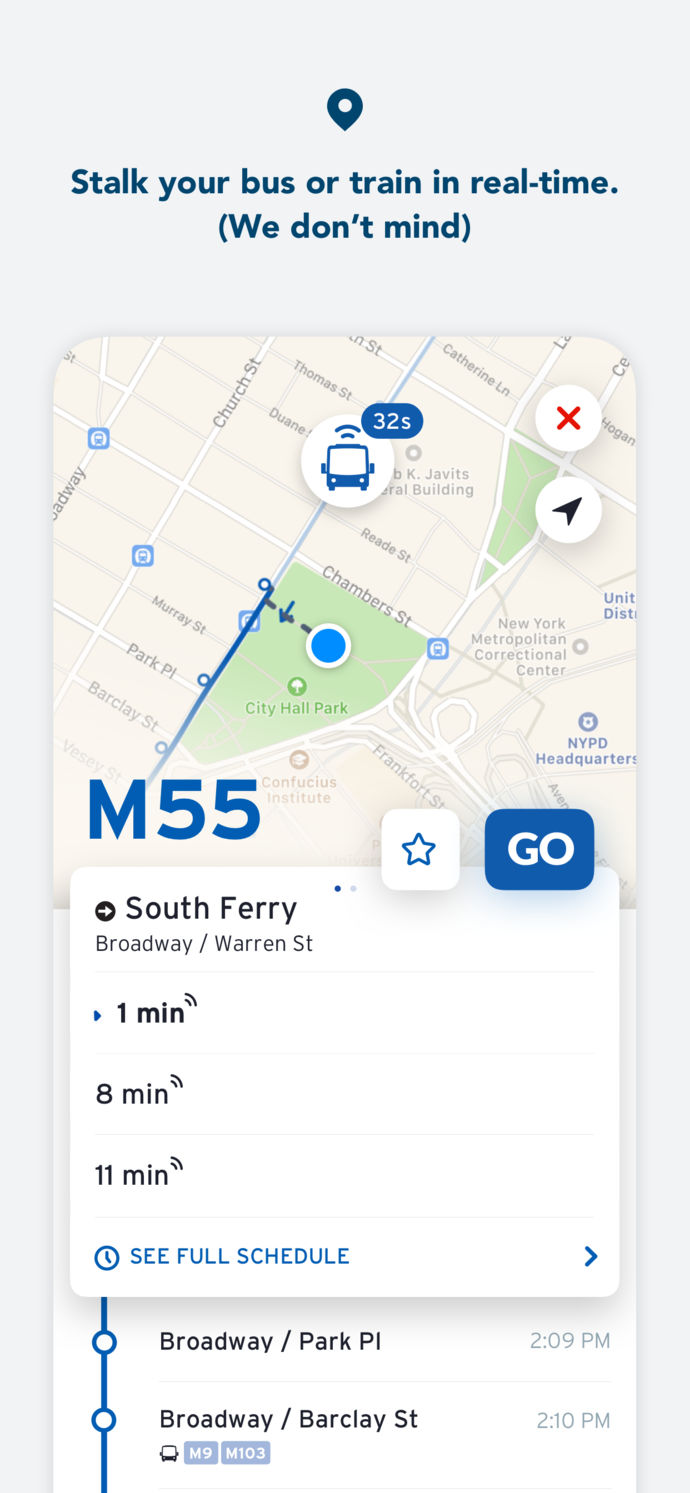This image is a detailed screenshot of a map application. At the very top, the heading is displayed in dark blue text, stating, "Track your bus or train in real time," accompanied by a humorous subtext in parentheses, "We don't mind." This suggests that the app provides real-time tracking features for public transportation.

Below the text, the map is prominently featured, showing real-time updates. Your current location is marked with a blue dot, while an icon of a bus is visible heading towards it. A timer next to the bus icon indicates that it is 32 seconds away from reaching you.

In the top-right corner of the image, there is an 'X' button, allowing users to close the screen, and a navigation button represented by an arrow pointing to the top right, typical of map apps for routing or direction purposes.

Towards the bottom left, the label "M55" identifies the specific bus or train line you are tracking. The bottom right corner features a "Go" button with a star icon to its left, possibly for marking favorite routes or destinations.

Additionally, the bottom part of the screen details the bus route, listing stops at "South Ferry," with estimated arrival times of 1 minute, 8 minutes, and 11 minutes for various points along the route. There is also an option to click "See full schedule" for a comprehensive view of the bus or train timings.